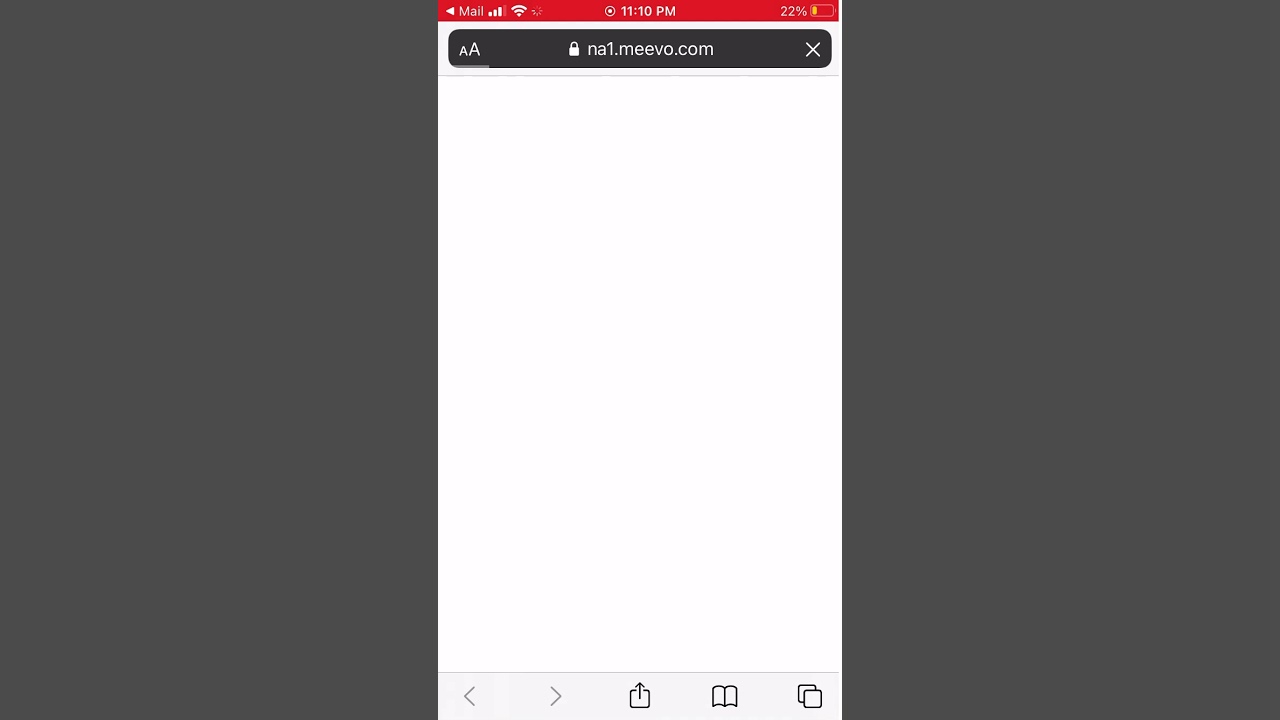The image showcases a computer or laptop screen displaying a screenshot of a smartphone interface. The image is in landscape orientation and is divided into three vertical sections. The left and right sections are plain dark gray, likely representing a background or placeholder surrounding the central content.

The central section features a bright white background, indicating the smartphone screen. At the top of this section, a prominent red bar spans the entire width. On this red bar, centralized white text reads "11:10 p.m.", with additional elements including a battery icon showing 27% charge on the right, and several other indicators on the left including an arrow, a partially obscured text likely indicating the carrier, a full signal bar, and a Wi-Fi icon.

Directly below the red bar is a thin white separator line under which lies a black bar also containing white text and icons, but with a white margin on either side. This bar includes a small 'A' next to a larger 'A' on the left (indicating text size adjustment options), a white 'X' on the right for closing, and in the center, a padlock icon followed by "na1.mevo.com," suggesting a website being viewed.

Further down, the main portion of the middle section is white, leading to a pale gray bar at the bottom, which contains navigation and action icons. These include left and right arrows for backward and forward navigation, an upload icon represented by a square with an upward pointing arrow, an open book icon, and an icon showing a piece of paper superimposed over another, perhaps indicating a multi-window or document function.